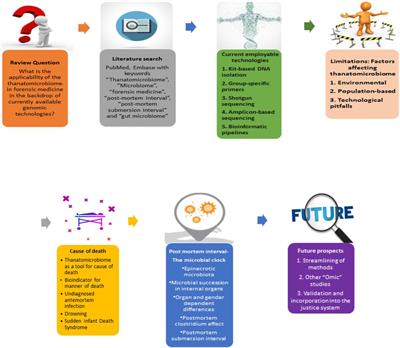The image is a detailed, colorful flow chart laid out on a white background, featuring seven distinct information fields, each highlighted in different colors and accompanied by unique icons. Starting at the top left, there's an orange square labeled "Review Questions," with black text and an icon of a person standing next to a question mark. An orange arrow then points to a gray box labeled "Literature Search," showcasing a camera icon. A blue arrow from there leads to a green box titled "Current Employable Technologies," featuring an icon of a partial human figure with hands spread out. This is followed by a green arrow pointing to a pink box (or beige in some descriptions) labeled "Limitations, Factors Affecting Ribosomes," adorned with an icon resembling a music note inside a circle with a human standing in the middle.

Continuing to the lower half of the image, a gray arrow labeled "Cause of Death" leads to a yellow box showing a hospital bed with a person sleeping on it, which is on wheels and purple in some descriptions. Next, a yellow arrow points to a blue box marked "Post Interview," which displays three yellow suns of varying sizes inside a gray circle. Finally, a blue arrow guides to the last box, a purple square labeled "Future Prospects," showing a magnifying glass with the word "future" written on it. Each of these elements is visually connected through arrows, forming a comprehensive flow chart that portrays a sequence of related steps or processes, though the exact nature of the chart remains somewhat unclear due to the tiny and hard-to-read text.